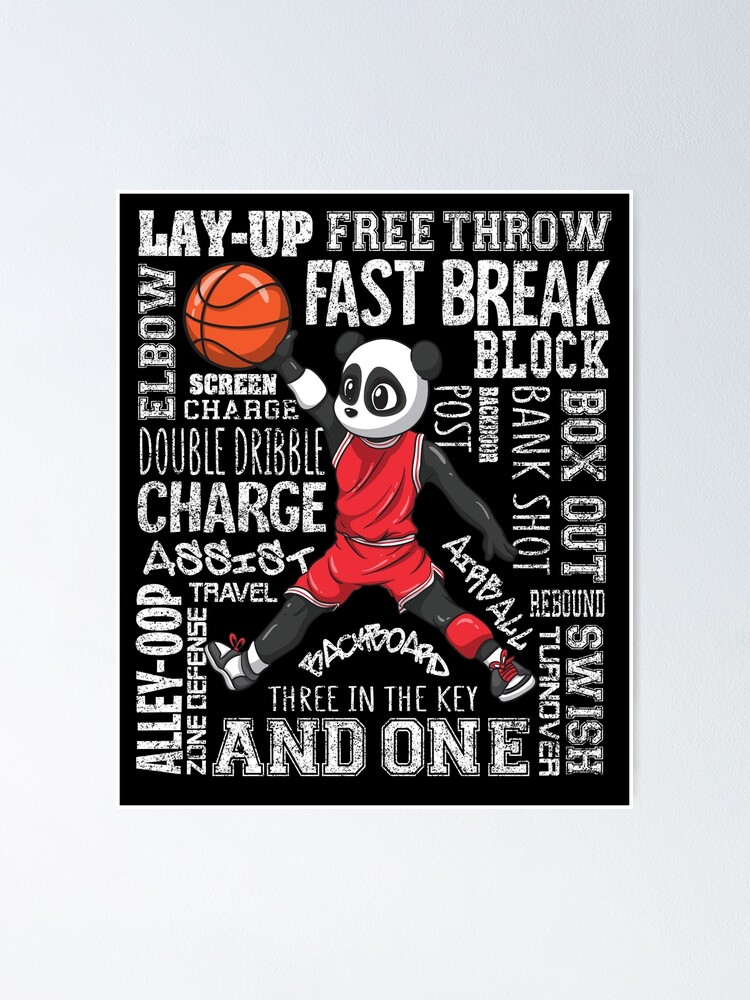The image is a detailed poster with a black background featuring a cartoon panda bear. The panda, depicted with large anime-style eyes, is dressed in a complete basketball outfit: a red sleeveless top with white trimming, matching red shorts, and grey and white basketball sneakers with red laces. Notably, the panda also wears a red knee brace on its left knee. The black and white bear, resembling a panda, is holding an orange basketball aloft in its right hand. The bear's fur is black on its arms and legs.

Surrounding the centrally placed panda are numerous basketball-related terms and commands in various fonts and sizes, all written in white. These terms include "Lay up," "Free throw," "Fast break," "Block," "Elbow," "Screen," "Charge" (written twice), "Box out," "Bank shot," "Post," "Double dribble," "Assist," "Alley-oop," "Zone defense," "Travel," "Backboard," "Airball," "Rebound," "Swish," "Turnover," "Three in the key," "And one," and "Back door." The text collectively emphasizes the theme of basketball, complementing the visual of the sporty panda bear. The panda’s black and white features contrast starkly against the dark background, making the vibrant colors and diverse text stand out prominently.